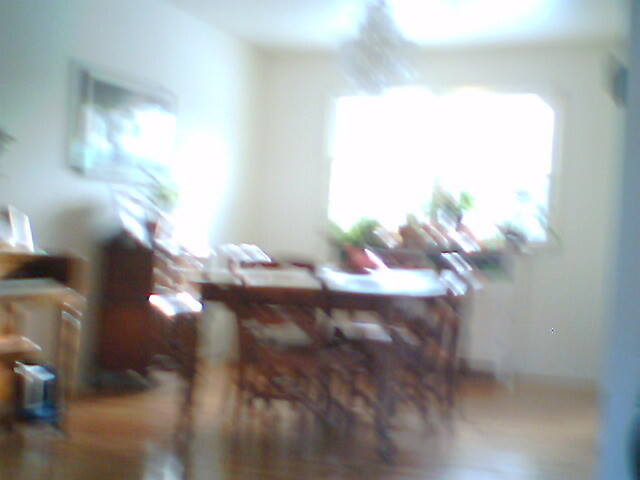The image is a blurry photo of a dining room taken while the camera was moving, causing multiple thin vertical lines. The central focal point is a dark brown wooden table surrounded by at least four chairs, situated on a lighter brown laminate floor. A plant is positioned on the table, adding a touch of greenery. Behind the table, a large rectangular window dominates the far wall, allowing daylight to flood the room and overexpose parts of the scene. The window's sill or a table beneath it holds additional plants in orange pots. A glass chandelier hangs above the dining table, further enhancing the room's ambiance. 

To the left, there is a small dark wood side table or dresser, possibly with another plant on top. Above this piece of furniture hangs a framed painting. Additionally, the left wall features a small, lighter-toned piano complete with a piano bench. The walls appear white, contributing to the room’s bright and airy feel despite the overall blurriness of the photograph.